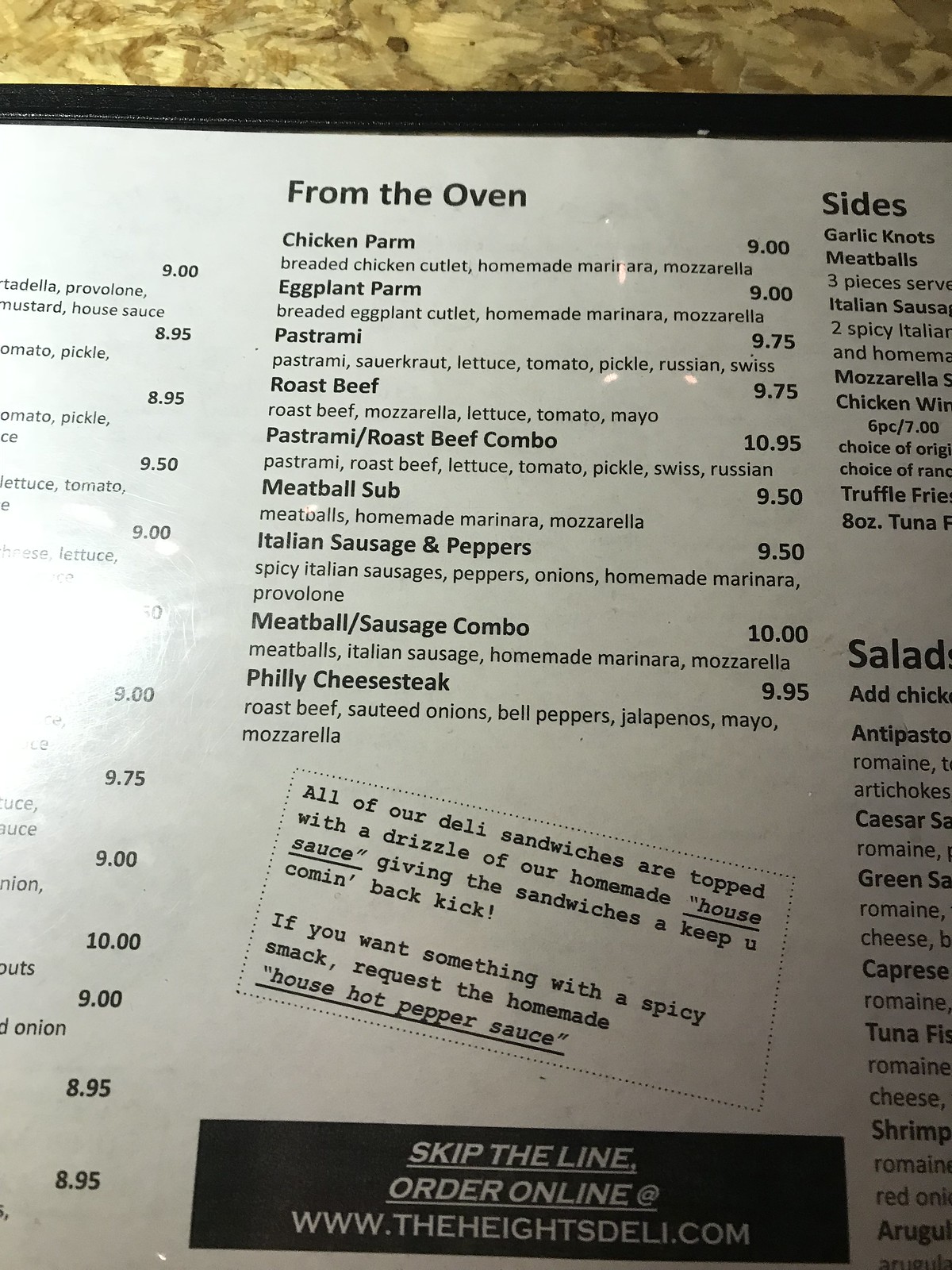This color photograph showcases a section of a restaurant menu placed on a table. The table, partially visible at the top of the image, features a light golden hue with black, gray, and brown marbling, resembling a luxurious marble surface. The menu itself is printed on white paper with black text. 

At the top-center of the menu, the header reads "From the Oven." Below this heading, several menu items are listed, including "Chicken Parm" (short for Parmesan), "Eggplant Parm," "Pastrami Roast Beef," "Pastrami Roast Beef Combo," "Meatball Sub," "Italian Sausage and Peppers," "Meatball Sausage Combo," and "Philly Cheesesteak." 

Near the bottom of the menu column, a black label with white text directs customers to "Skip the line, order online," followed by the website www.theheightdeli.com. Just above this label, there is a sideways slip of paper that reads, "All of our deli sandwiches are topped with a drizzle of homemade house sauce, giving the sandwiches a keep-it-coming-back kick."